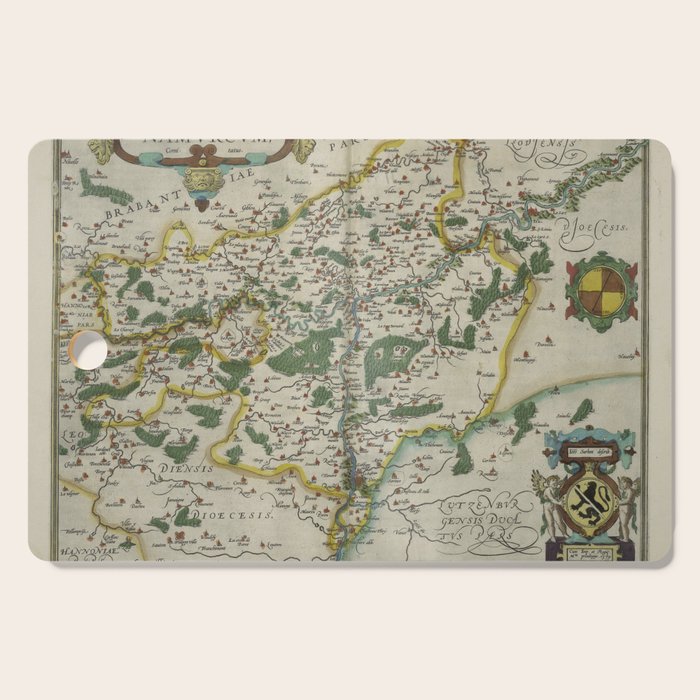This image depicts an intricately detailed, ancient map print that resembles an old, fable-like map you might find in a classic book. The background is an ivory color, and the map is adorned with various colors, prominently featuring highlights in green and yellow, with some dark brown elements adding depth. A noticeable crease down the middle suggests this print is part of an open book. At the bottom of the map, there is a chest of arms flanked by two angels who appear to be holding a lion. The map is filled with numerous names and places in fancy, difficult-to-read script, including "DIENSIS" and "DIOECESIS." Wavy yellow rivers and lush green trees are depicted across the map’s landscape, adding to its rich, historical feel. Fancy writing and other detailed, intricate designs further embellish the map, enhancing its antiquated charm.